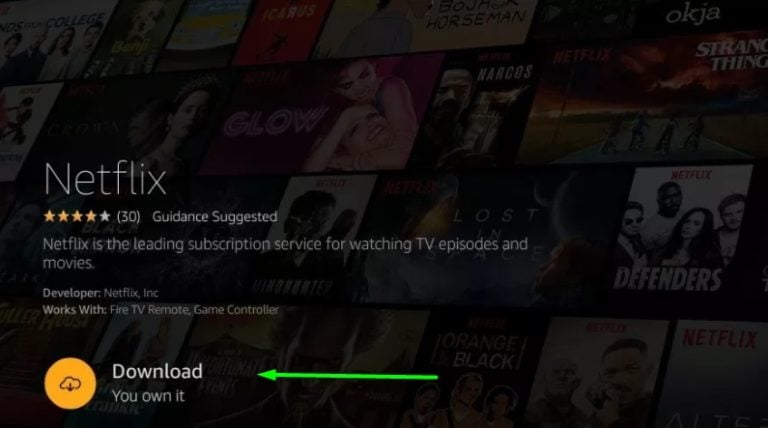This screenshot captures the interface of the Netflix app or website. Prominently positioned on the far middle left is the Netflix logo in white text. Below this, review ratings are displayed, showing a current rating of four out of five stars with the first four stars colored in gold and the last one in silver. Adjacent to this rating, the number 30 is enclosed in parentheses, indicating the number of reviews. Next to the review count, the phrase "Guidance Suggested" is mentioned, possibly referring to content advisory.

The description under the ratings reads, "Netflix is the leading subscription service for watching TV episodes and movies." Following this, the developer is listed as "Netflix Inc." Further information specifies compatibility, noting it "works with Fire TV remote and game controller". 

In the bottom left corner, there is a circular icon featuring a cloud symbol with the word "Download" beside it, and beneath this, the message "You own it." Towards the bottom middle, a green arrow points to the word "Download," emphasizing the download option.

The background showcases a selection of popular movies and TV shows arranged side by side, including titles like "Glow," "Defenders," and "Stranger Things," enhancing the visual appeal of the interface.